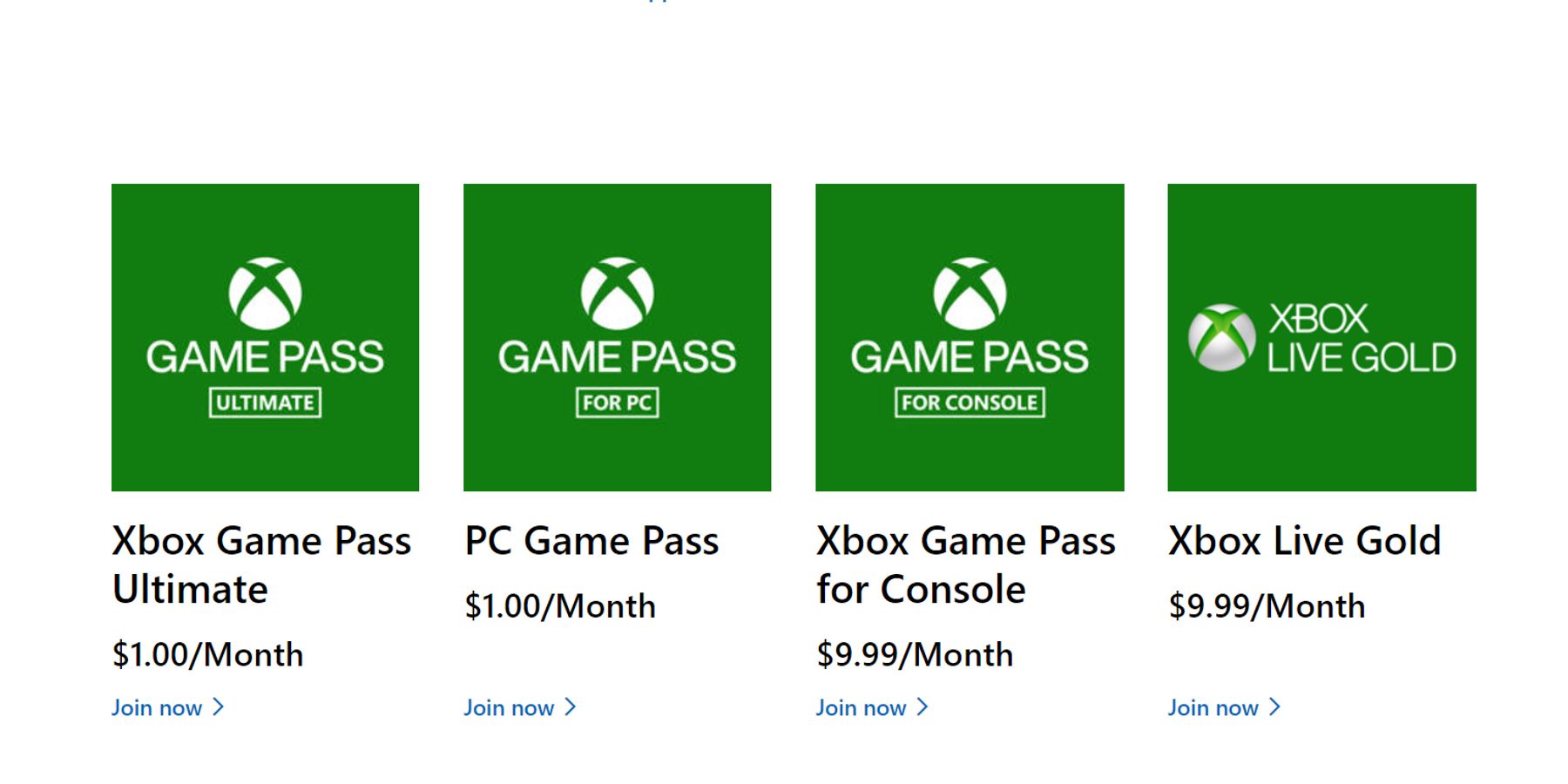This image displays four Xbox game subscription options against a white background. The options are presented side by side, featuring green boxes. 

1. **Game Pass Ultimate**: At the top, there's an Xbox icon. The text reads "Xbox Game Pass Ultimate" with a price of "$1/month" followed by a blue "Join Now" button.
  
2. **Game Pass for PC**: Similar to the first, this option has the Xbox icon and the text "Game Pass for PC" with "$1/month" in black, accompanied by a blue "Join Now" button.

3. **Game Pass for Console**: This box also sports the Xbox icon. It reads "Xbox Game Pass for Console" with a price of "$9.99/month" and includes a blue "Join Now" button underneath.

4. **Xbox Live Gold**: This differs slightly with a circle icon featuring a green section. The text states "Xbox Live Gold" priced at "$9.99/month," with a blue "Join Now" button below.